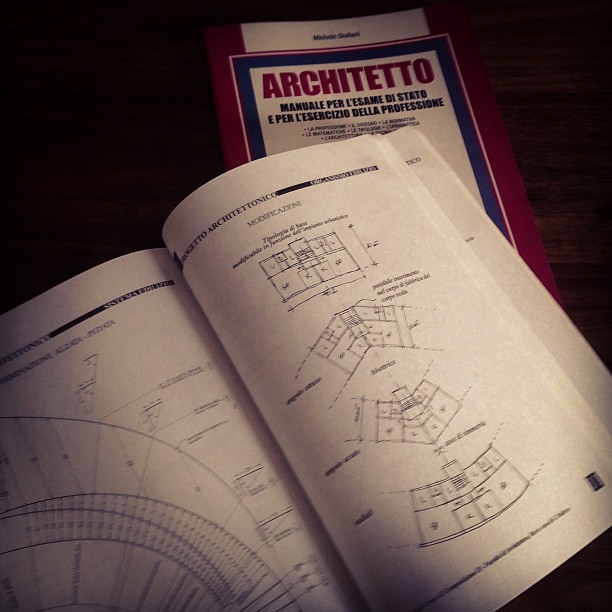The image showcases an open architectural manual with white pages and intricate black diagrams, likely of various beams or material sections, detailing dimensions and angles. The diagrams feature lines crisscrossing in multiple directions, making the text difficult to decipher due to its small size. In the background, under a shadowed dark brown surface, lies a closed book with a red, white, and blue cover. The title of this secondary book is displayed prominently in red letters and appears to read "Architetto," suggesting it is an architectural book in Italian. The contrasting colors and detailed drawings create a focused scene of architectural study and reference.